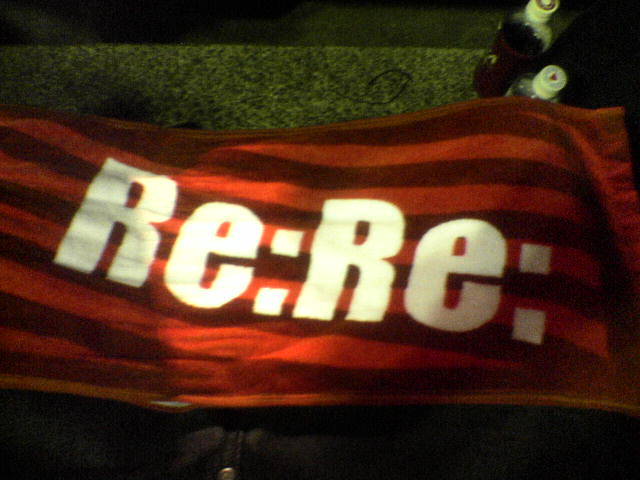This square image predominantly features a red banner with dark red horizontal stripes across it. The banner, centered horizontally and taking up about two-thirds of the middle section, displays large white block text that reads: "RE:RE:". The text alternates with capital letters (R and E) and colons, evoking the format of responses in email threads.

The banner appears to be lying on a dark gray granite surface, which is partially visible. Above the banner, in the top right corner, stand two bottles filled with dark liquid, each capped with white lids. The scene is further complemented by hints of green grass visible in the background, suggesting an outdoor setting. Adding depth to the image, there is some kind of black fabric with a button that subtly peeks out from the lower portion, left of center – potentially hinting at a pair of jeans or another textile just at the edge of the frame. The overall style of the photo suggests that it was taken from above, possibly as a casual snapshot, given its slightly dark and blurry characteristics.